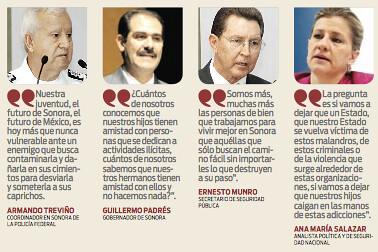The image is a color clipping from a Spanish magazine or newspaper featuring quotes from four distinct individuals. Each person is showcased in a vertical column with their photograph, a quote, and their name beneath it, highlighted in burgundy. The first column features an elderly man with white hair, standing in front of two small black microphones and wearing a uniform, all set against a tan background. He looks away to the right, and his quote is marked by large burgundy quotation marks, with his name in the same color. The second column displays a light-skinned man with dark hair, a receding hairline, and a black mustache, dressed in a suit. The third column also shows a man, this time with dark brown hair, wearing wire-rimmed glasses and a light-colored shirt paired with a black jacket. The fourth column features a woman with white skin and blonde hair pulled back, adorned in a dark pink suit and earrings. Each quote is emphasized with red quotation marks, followed by the individual's name and possibly their job title in black text.